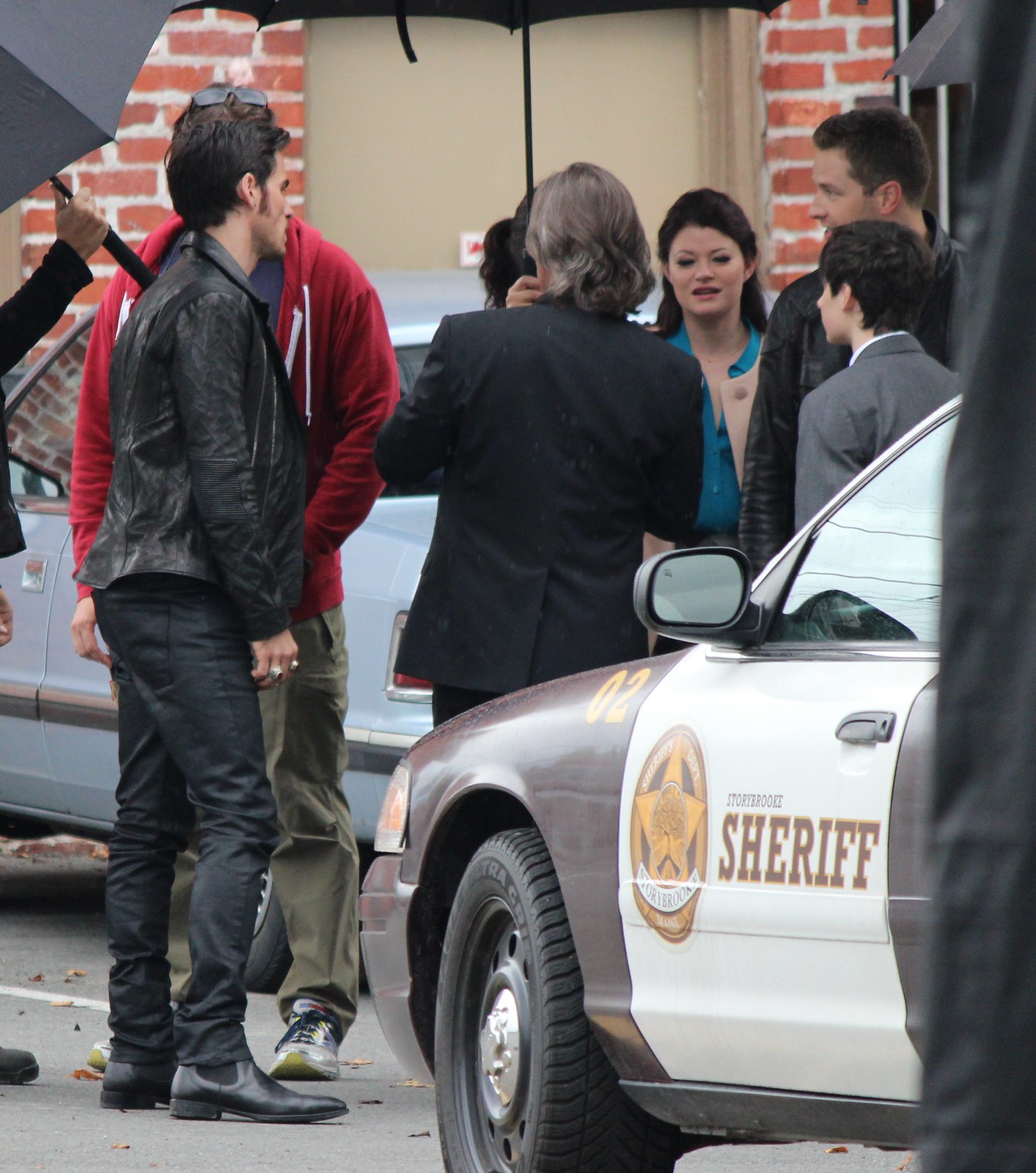This photo captures an outdoor scene likely from a movie or TV set, where a diverse group of people is gathered in a circle. Dominating the left of the image is a sheriff's car emblazoned with "Storybrooke Sheriff" on its side. The group, composed predominantly of white individuals across various age ranges, includes a younger boy, middle-aged men and women, and younger adults in their 20s and 30s. Many of them are actors, identifiable by stagehands holding black umbrellas over them. On the left side of the picture, a man in his early 30s with medium black hair is dressed entirely in black leather, complete with a leather jacket, pants, and cowboy boots. Next to him stands another man wearing a red sweatshirt with a white zipper and green pants. Central in the frame is a man in a black suit with long black and gray hair and a woman facing the camera with long black hair. The setting appears to include another partially visible blue car and part of a red brick building in the background, rounding out this vibrant behind-the-scenes snapshot.